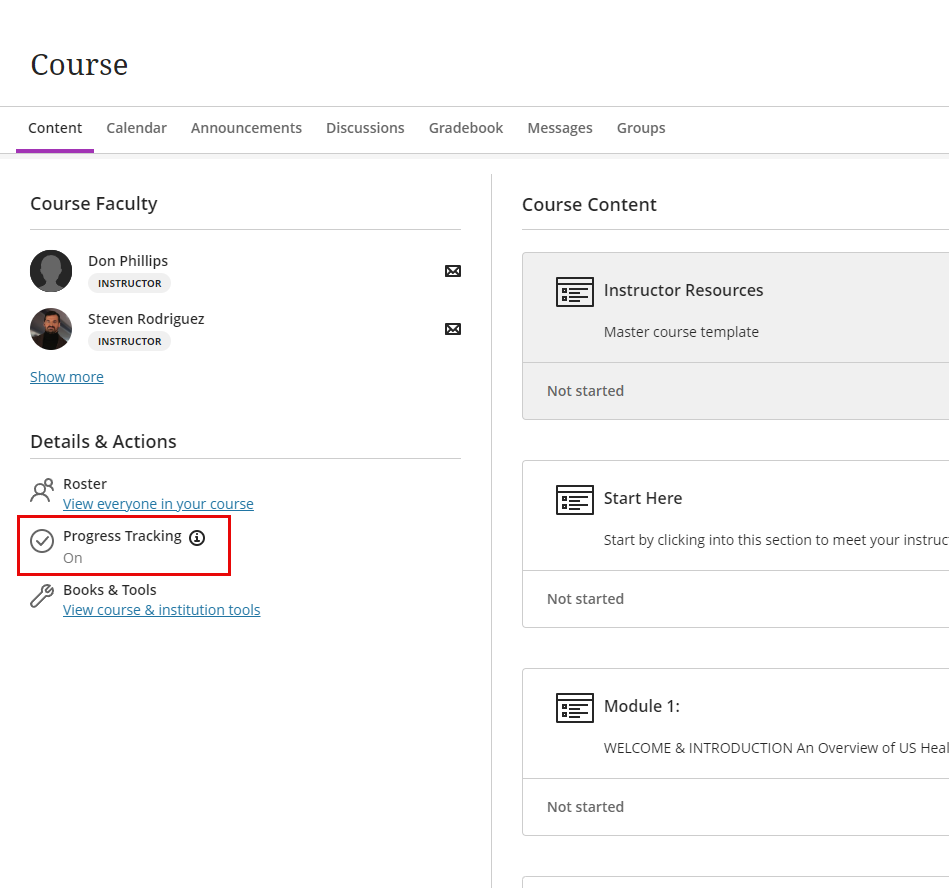**Detailed Caption for Screenshot:**

The image is a landscape-oriented screenshot of an online course platform's interface. The creator of the screenshot has highlighted a specific section with a vibrant red triangle and a red rectangle to draw attention.

In the upper left-hand corner of the interface, there is a navigational menu. The first row of this menu is labeled "Course." Beneath it, subsequent rows list options as follows: Content, Calendar, Announcements, Discussions, Gradebook, Messages, and Groups. The "Content" section is highlighted with a purple stripe beneath it and is in bold font, indicating the user is currently on the 'Content' page.

The 'Content' page is divided into two main columns. In the top left of the first column, there is a heading "Course Faculty." Under this heading, two instructors are listed: Don Phillips and Stephen Rodriguez, with Stephen Rodriguez's name accompanied by a small image of his portrait. Directly below Stephen Rodriguez's name, there is a clickable link labeled "Show More" that likely expands to display additional information about the instructors.

Further down in the first column, another section titled "Details and Actions" can be seen, followed by "Roster" with a live link labeled "View everyone in your course." The red rectangle highlights a particular area that specifies "Progress Tracking: On," indicating that the current user has activated progress tracking for the course. Below this highlighted segment, there is another section titled "Books and Tools" with a link prompting the user to "View course and institution tools."

The right column is labeled "Course Content." Underneath this label, there is a gray box with the text "Instructor Resources: Master Course Template - Not Started." Following this section, another block titled "Start Here" invites users to begin by clicking into the section to meet the instructor. As we proceed down the column, other sections appear but are cut off towards the right-hand side of the screen. These sections are titled "Module One: Welcome and Introduction," and "An Overview of US Health" which is followed by the note "Not Started," but both lines are partially obscured.